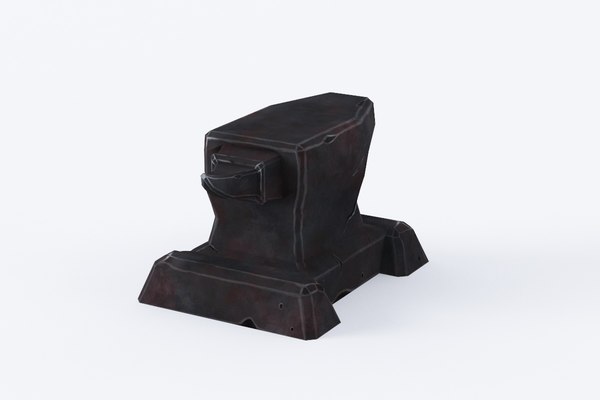The image is a detailed, photographic representation of a black anvil placed against a clean, white background. The anvil is oriented at a slight diagonal angle with its pointed protrusion—resembling a horn—facing the camera. The construction of the anvil consists of a black base comprised of two leg-like components connected by a central member, supporting the main anvil body. The anvil itself starts low, tapers inward, and then flares outward, resembling a stylized coffin shape, particularly at the top. Light reflects off the anvil's edges, creating white highlights that add to the definition of its shape. A subtle shadow is cast to the right of the anvil, suggesting a light source from the left side. The overall image is devoid of any text or additional elements, focusing entirely on the striking contrast between the dark anvil and the pristine background.